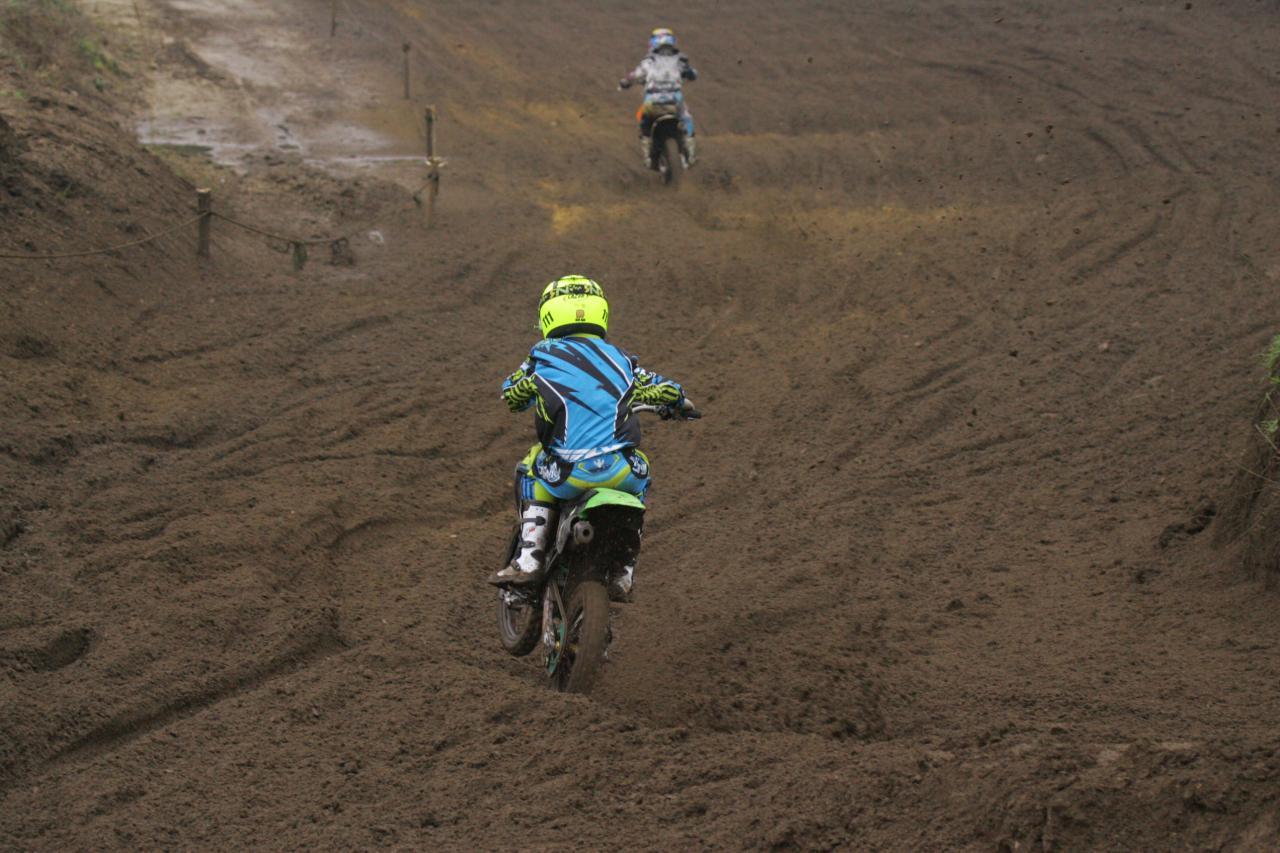This image captures a vibrant, outdoor scene during daylight of two kids riding dirt bikes on a well-worn, loose dirt track. The foreground features numerous tire marks and small hills, with a predominantly brown, dirt-covered ground. Along the left edge of the image, a boundary marked by a series of small wooden posts connected by ropes is visible. The nearest rider is centrally placed, wearing a bright, neon yellow helmet, blue and black outfit, and white-detailed black boots. His dirt bike has a bright neon green fender. Behind him, another rider, farther in the distance, sports a blue helmet and a white jersey speckled with either dirt or black dots. The entire scene suggests an outdoor dirt bike track, with both children riding away from the viewer, and the overall setting bathed in natural daylight.